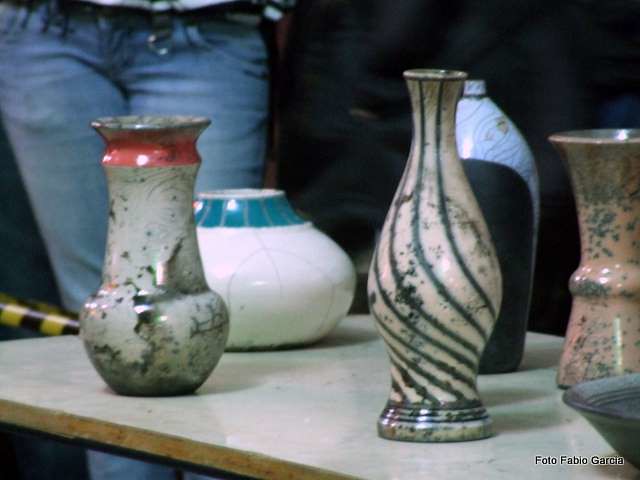The image captures a display of five distinct ceramic vases and a small metal bowl arranged on a white stone table. The vases in the foreground exhibit a range of hues and details: the first on the far left is pale green with darker hues bleeding in and a reddish dark pink lip, characterized by its rounded bottom narrowing into a thin neck. Directly behind it, a large vase with a wide bottom and sharp slant upward shows a dark teal neck and a body adorned with black lines on white. In the center, the tallest vase thins out at the base, widens in the middle, then slants up to a light tan finish with black specks and lines. Next, a short, thick black vase with a very small opening displays blue near the top and a black band around its neck. On the far right, a plain tan and pink vase with dark green speckles around the neck widens slightly at the top, thins out, then flares into a wide opening. A small metal bowl sits just visible at the bottom right, above the "Photo Fabio Garcia" brand. A figure in light blue denim jeans stands behind the table, partially hidden by a dark backdrop and potentially a yellow and black barrier stripe.